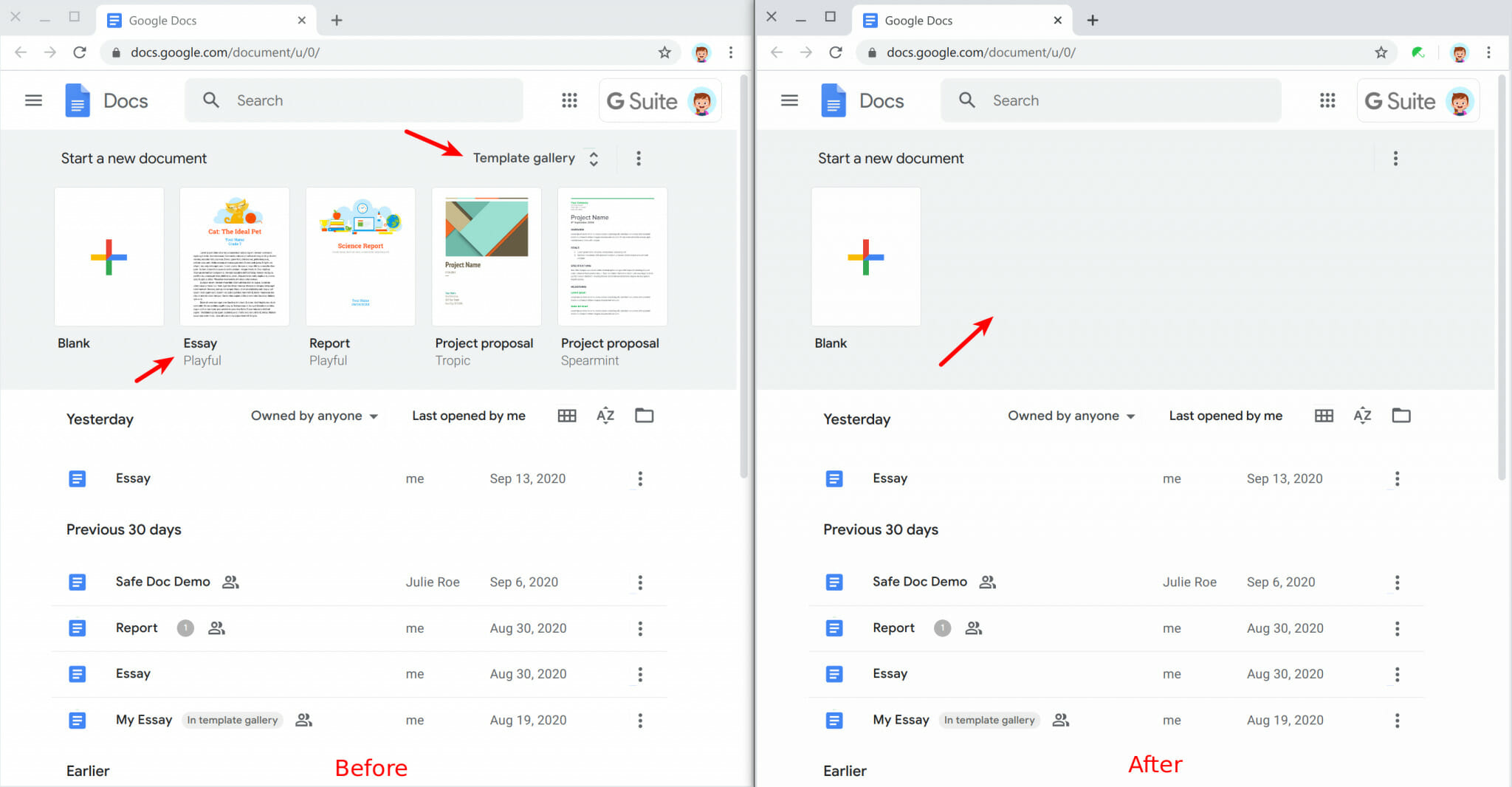The image is a screenshot of a Google Docs interface. The URL displayed at the top is "docs.google.com/document/u/0/". The primary content shown includes:

1. A digital representation of a blank page.
2. An essay titled "Playful," accompanied by a picture of a cat next to a large red yarn ball. 
3. Another essay titled "Cat, the Ideal Pet," categorized as a science report.
4. A project proposal.
5. A second project proposal named "Spearmint."

Additionally, there are document details indicating activity status:
- "Last Opened by Me, September 13, 2020, Previous 30 Days"
- "Safe Doc Demo, Last Opened by Julie Rowe, September 6, 2020"
- "Report Last Opened by Me, August 30, 2020"